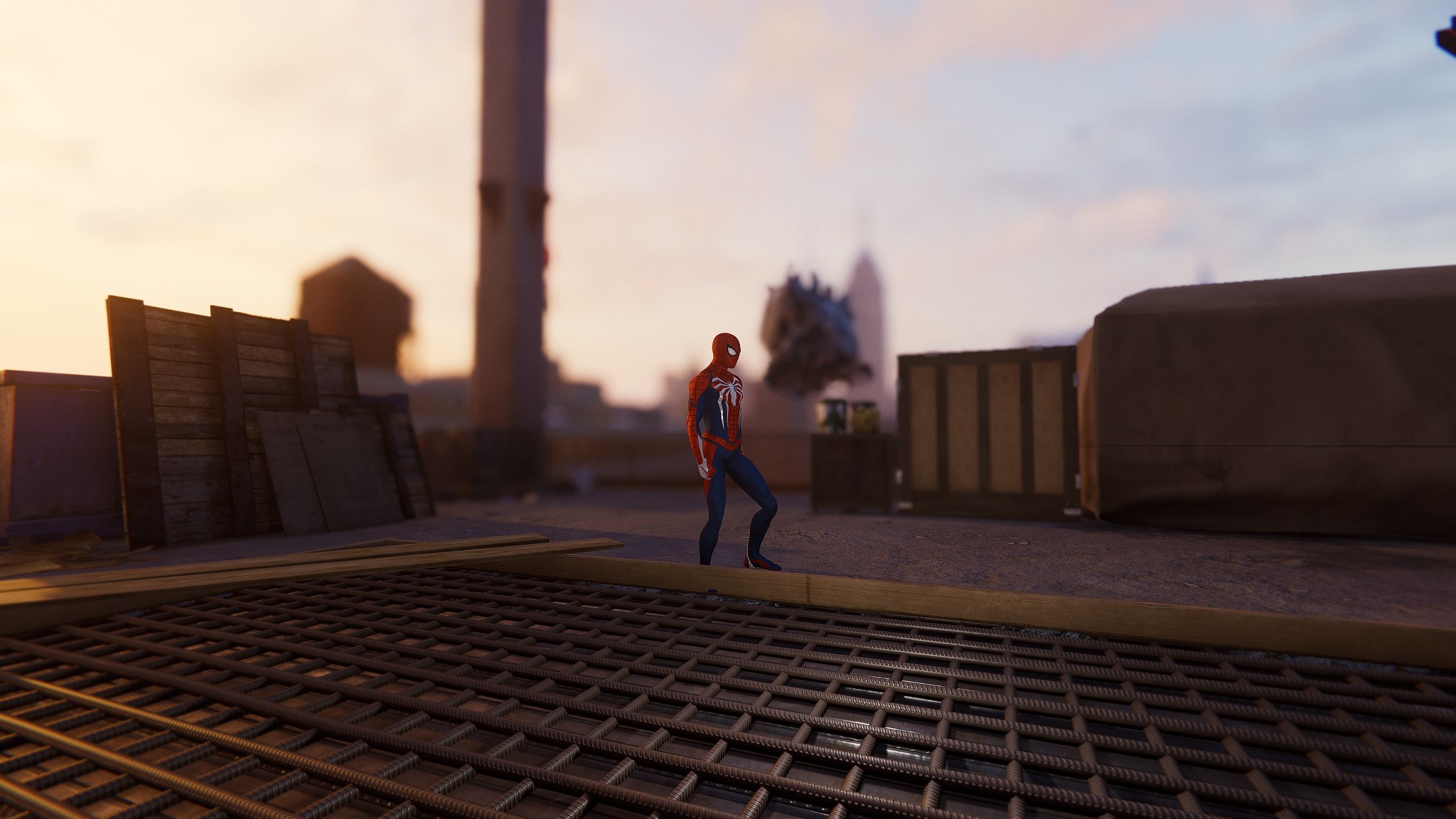A high-resolution image from a modern Spider-Man video game, likely Spider-Man 1 or 2 on the PlayStation 4 or 5, showcases Spider-Man in his classic red and blue suit. He stands prominently at the center, adorned in blue pants and a red torso, with red extending down his arms and blue side accents. A large, bright white spider emblem decorates the middle of his chest, and his iconic red mask features stark white eyes. The setting appears to be a rooftop, featuring a textured, black rebar-like floor. To the side, pallets can be seen, indicating a construction site or storage area. The background displays a partly cloudy sky with shades of blue and white, and a smokestack or pillar adds to the urban rooftop ambiance.